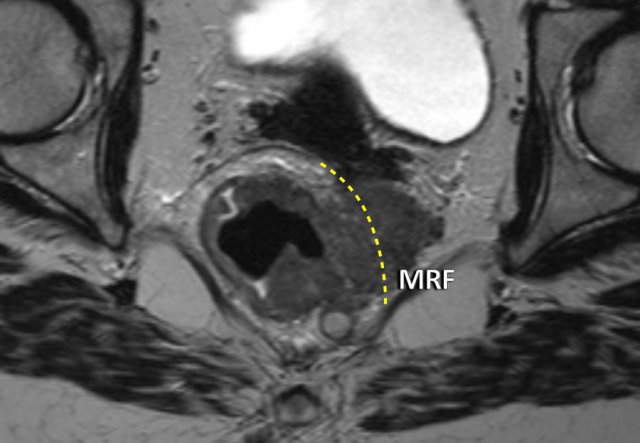The image appears to be a detailed black-and-white MRI scan of a person's head. Dominating the top center is a white, bean-shaped blob outlined in black. Below this blob, a dark, cloud-like formation extends downward and is flanked by transparent, liquid-like areas. In the center of the scan, slightly left of the midpoint, there's a distinct circular object with a darker core. Adjacent to this, a series of short, dashed yellow lines arc in a downward-right direction from roughly the 12 o'clock to 4 o'clock positions. To the right of these lines, in bold white letters, it reads "MRF." Surrounding this central area, intricate strands of black chords, resembling intertwined strands, stretch out towards the left and right upper corners of the image, as well as the lower corners, creating a mirrored, symmetrical pattern. The whole image measures approximately five inches wide by three inches tall and contains intricate variations of gray and black tones.